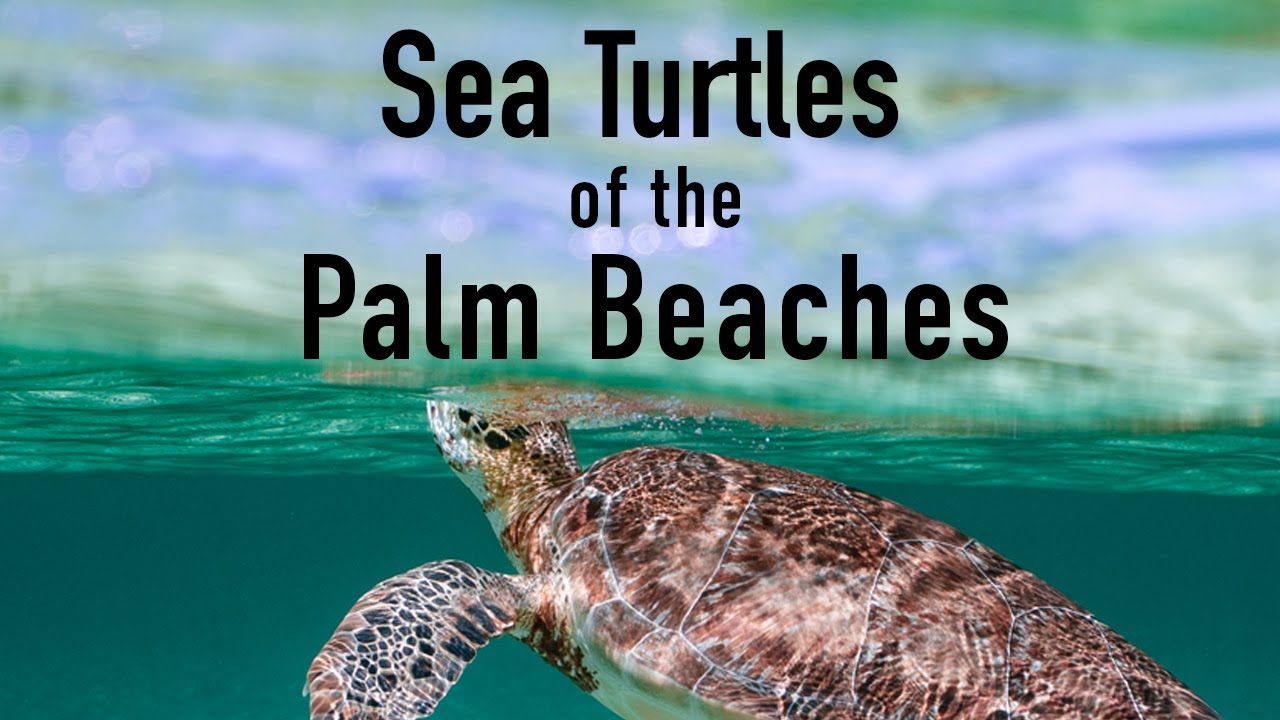The photograph captures a close-up of aquamarine sea water with shimmering, blurry shades of blue and green on its surface. Swimming just below the waterline, a medium-sized sea turtle with a brown and black patterned shell and similarly colored skin is seen. The turtle is propelling itself upwards with its flippers, and its head is partially emerged from the water surface, revealing a dark black eye and a whitish chin. The background is a blend of indistinct shades of green, blue, and white, possibly hinting at a distant resort. The image is brightly lit by sunlight, enhancing the vibrant colors. Text overlaying the top of the image reads, "Sea Turtles of the Palm Beaches."